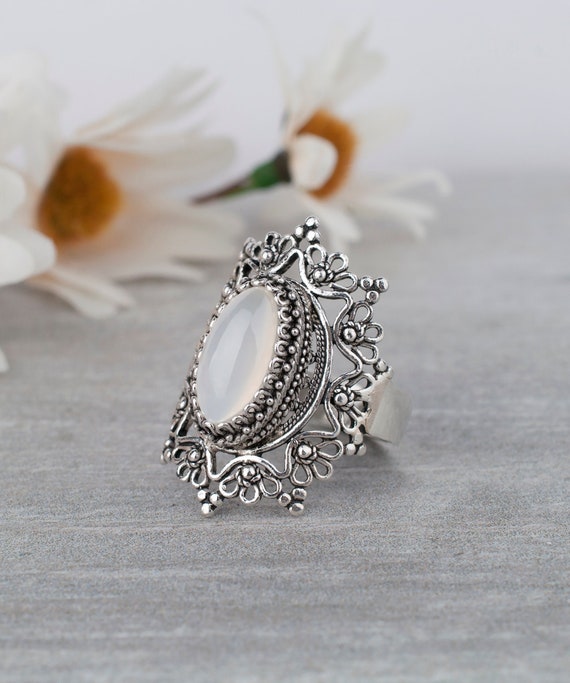In the foreground of this advertisement image, a meticulously crafted silver ring rests on a smooth gray surface that mimics faux wood. The ring, which appears to be rounded but slightly oval in shape, boasts a thick band and ornate design that encompasses intricate, swirling floral patterns. At its center, cradled by these delicate silver arches and small reflective spheres, lies a clear, milky white gem. This semi-transparent jewel is encircled by a reflective silver wreath, resembling sunbeams radiating outward. In the out-of-focus background, against a white wall, two white-petaled flowers with vibrant orange-yellow centers and green stems add a soft contrast, reinforcing the elegance of the scene. The overall setting gives a timeless, almost heirloom-like quality to the ring, though it could also serve as an exquisite piece of costume jewelry.